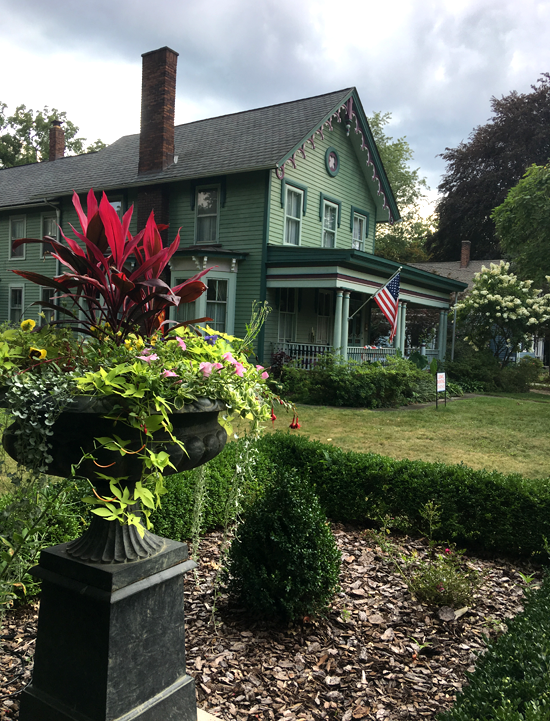This outdoor photograph features a charming colonial-style, two-story house painted in green with dark green window trims and a grey sloping roof. Prominently displayed in front is an American flag, emphasizing the home's traditional American character. The house is surrounded by lush greenery, including trees with vibrant green leaves, a white flowering tree or shrub to the right, and neatly trimmed dark green hedges. 

In the foreground on the left, there is a beautifully adorned stone flower pot bursting with colorful plants, featuring a striking maroon or red plant in the center surrounded by green vines and flowers. This meticulously maintained garden adds to the picturesque setting. There is also a black, memorial-like stand holding additional flowers, contributing to the ornate landscaping. The entire scene is captured in daylight, showcasing the detailed architecture and vibrant garden in all its glory.